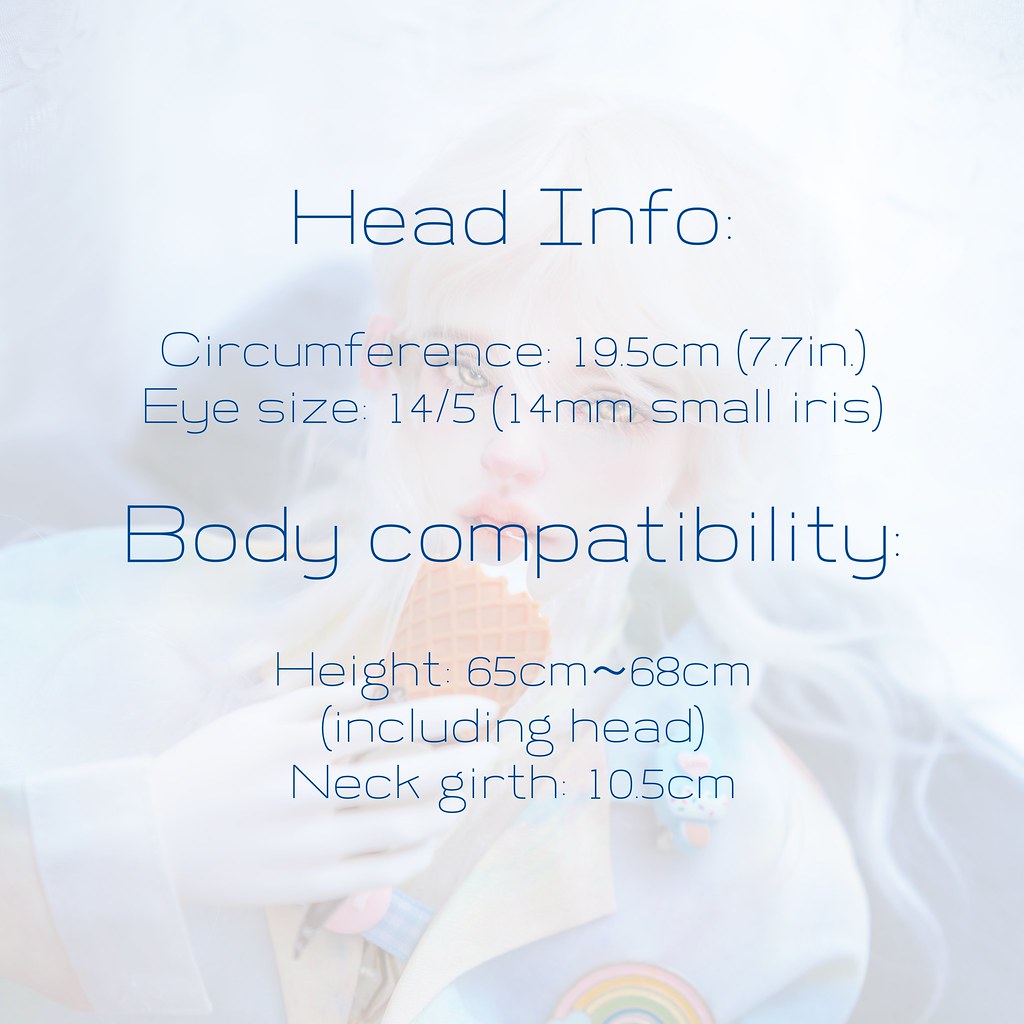The image is a tall, rectangular advertisement that faintly depicts a young woman licking a light brown ice cream cone and looking directly at the camera. The background is primarily white with a subtle blue overtone. The woman has long, silvery-blonde hair flowing towards the bottom right corner and is colored very pale. She has a pink nose and pink lips. She is wearing a blue jacket with a white collar and a rainbow logo on the left breast, featuring colors like orange, yellow, pink, blue, and green. The woman's hand emerges from the left corner, holding the ice cream cone to her mouth. The image is overlaid with thin blue text that reads: "Head info: circumference 19.5 centimeters (7.7 inches), eye size 14/5 (14 mm, small iris). Body compatibility: height 65 centimeters ~ 68 centimeters (including head), neck girth 10.5 centimeters."